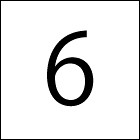The image showcases a simple yet striking design: a small, white square bordered by thin black lines, creating a minimalist frame. Inside this bordered square lies a prominent, thick black number six, centered perfectly. The square forms four precise right angles, enclosing the stark contrast of the heavy black numeral against the clean white interior. The number six, defined by a solid, thick stroke, features an oval-shaped loop at the top. This black-and-white image is devoid of any photographic elements, text, people, animals, plants, buildings, or mechanical objects, emphasizing the bold graphic design of the central number within its precise geometric border.